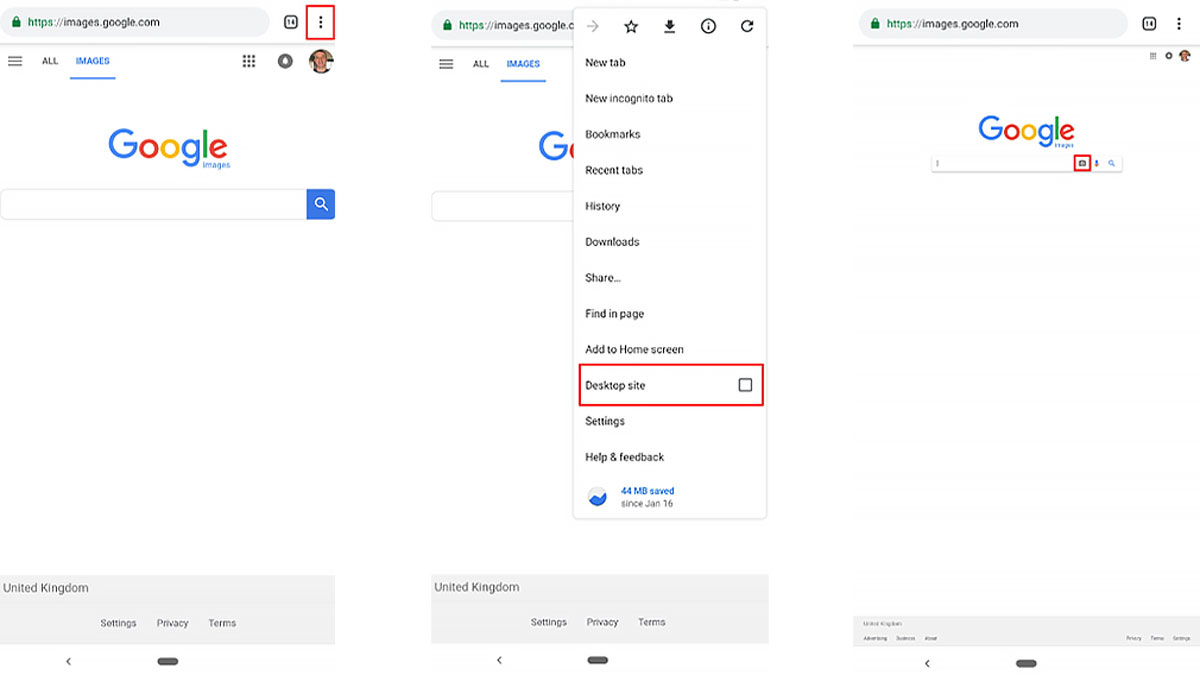The image is a step-by-step guide for accessing the desktop version of Google Images on a mobile device. The sequence consists of three screens:

1. The first screen shows the Google Images homepage (images.google.com) in the address bar.
2. The second screen displays the browser's menu, indicated by three vertically stacked dots in the top right corner. This screen has a red box highlighting this menu icon, which has been clicked to reveal a dropdown menu.
3. The third screen illustrates the expanded dropdown menu with an emphasis on the "Desktop site" option, marked by a red rectangle around it. Additionally, a red box highlights a small black square icon with a white center on the Google Images homepage, suggesting it might be an important feature or tool in the desktop interface.

This guide would assist users in switching to the desktop site view on their mobile browser to access potential additional functionality or a different user interface on the Google Images platform.